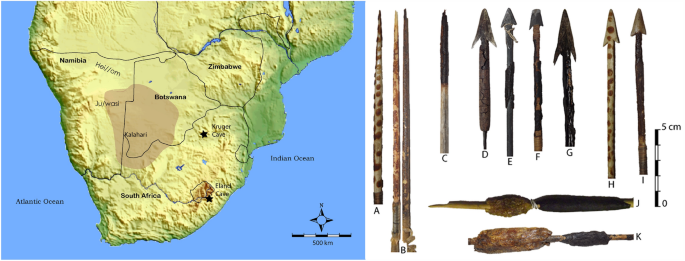This graphic, oriented in landscape, is divided into two sections, each containing a detailed landscape image. The left section features a map of the southern part of Africa, depicting countries such as South Africa, Namibia, Botswana, and Zimbabwe. The terrain is illustrated with a textured green and brown background, indicative of varying altitudes, with green for low areas and yellow for highlands, alongside black borders delineating country boundaries. The map also highlights significant locations like the Kruger Cave and the Elinor Cave in South Africa, marked with black stars. Bodies of water include the Atlantic Ocean on the left and the Indian Ocean on the right, rendered in light blue. Additional map elements include a compass for orientation, and a scale denoting 500 kilometers. 

The right section of the graphic showcases an array of primitive tools set against a white background. These tools, resembling spearheads and daggers of various shapes and sizes, appear weathered and ancient, suggesting they were excavated from archaeological sites. Their lengths are indicated by a scale from 0 to 5 centimeters, revealing most tools exceed this measurement. The tools are cataloged with labels ranging sequentially from A to K, emphasizing their order and variety.